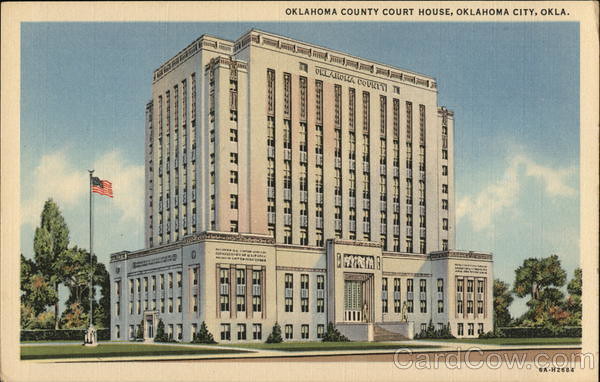The image is a scanned photograph of a vintage postcard depicting the Oklahoma County Courthouse in Oklahoma City, Oklahoma. Encased in a slightly discolored tan border, the dimensions of the image appear to be approximately three inches high by six inches wide. The top right corner of this border bears the caption "Oklahoma County Courthouse, Oklahoma City, Okla." in black text, while the bottom right reads "GAH2686." A semi-transparent watermark stating "cardcow.com" is superimposed over the entire image.

The central illustration reveals a large, rectangular, multi-story white courthouse with classical architectural elements. The base of the building spans three stories and features a grand entrance with steps flanked by statues, leading up to the doorway. Extending upward from the center base, a tall tower of additional stories rises, giving the structure a distinctive profile. The building's facade is characterized by numerous windows.

In the background, blue skies with clouds create a pleasant ambiance, complemented by green grass and a few trees on either side of the courthouse. Prominently on the left side of the image stands a flagpole flying the American flag, adding a patriotic touch to this detailed artistic rendition.